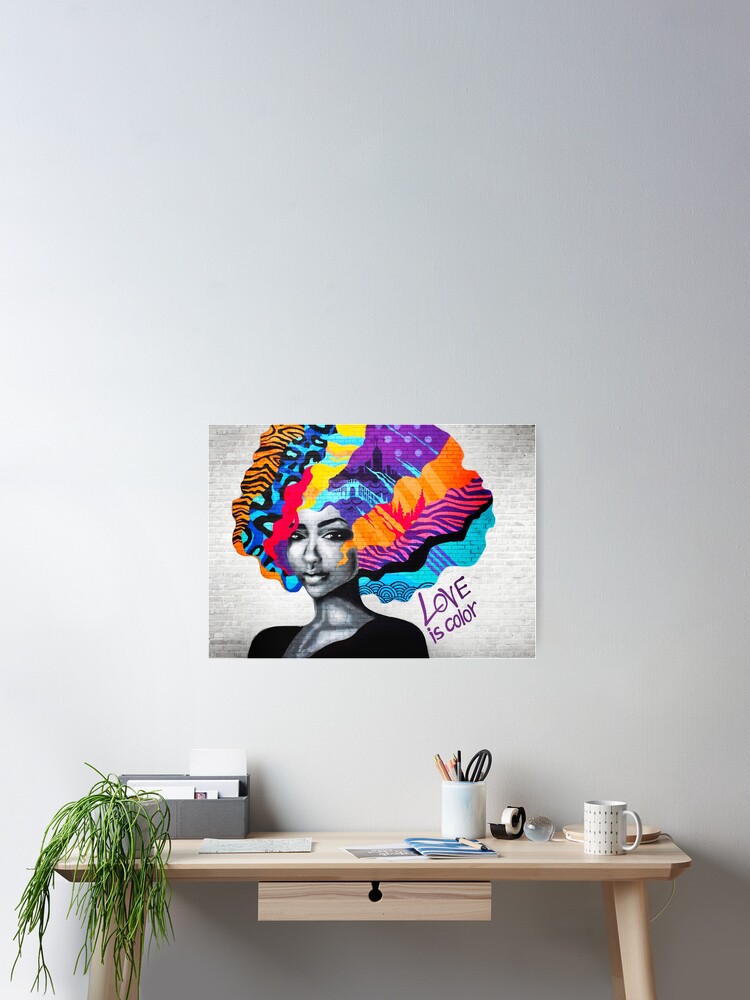In the room, a tall white wall serves as the backdrop for a striking poster. The poster features a black and white portrait of an African American woman with a multitude of multicolored, patterned streaks in her hair, including hues like purple, orange, blue, red, yellow, and pink. She wears a black top and stands against a grey, brick-patterned background. Next to her, the words "Love is a Color" are prominently displayed in purple. Below this vibrant artwork, a light brown, possibly whitewashed wood desk with a central drawer is situated. The desk is seen from the side, showing miscellaneous items arranged on its surface: a lamp that leans over to the right, a small flower pot with green leaves cascading over the left edge, a cup brimming with scissors, pencils, and pens, a tape dispenser, a white cup with a design, various papers, and additional stationery. On the far left, a holder contains white items, completing the functional yet decorative arrangement.